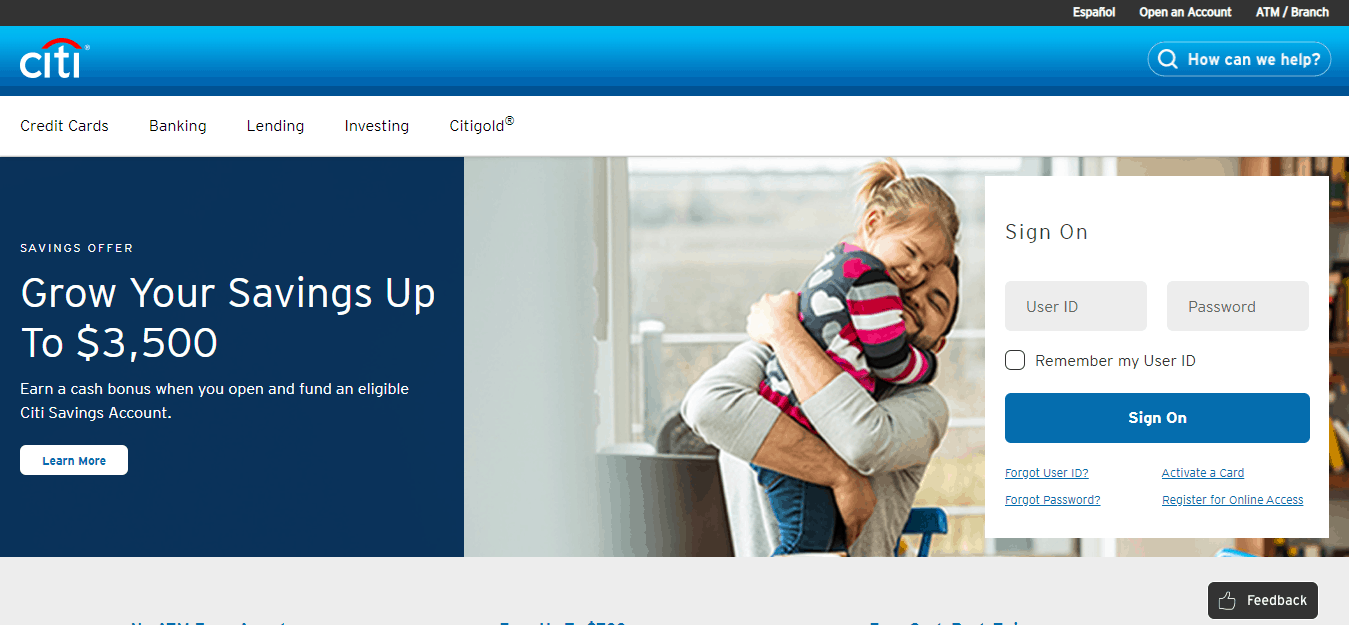The image depicts a partial screenshot of the desktop version of the CitiBank website. The top of the image features a horizontal blue navigation bar. On the far left of this bar, the "Citi" logo is clearly visible. At the far right end, there is a button labeled "How can we help?" Directly above this button, there's a compact menu with the options "Español," "Open an account," and "ATM/Branch."

Below this navigation bar, and aligned to the left, is a dark blue square containing a white text announcement: "Savings Offer - Grow your savings up to $3,500. Earn a cash bonus when you open and fund an eligible Citi savings account." Accompanying this message is a "Learn more" button for additional details.

To the right of the promotional message, there is an image of a smiling man lifting and holding a young girl, both appearing joyful.

Overlapping the right side of the image is a typical login section in a white square. It includes fields for "User ID" and "Password," along with a checkbox option labeled "Remember my User ID." Directly below these fields is a blue "Sign On" button. Underneath the 'Sign On' button, there are four links, although only "Forgot User ID" and "Forgot Password" are legible, while the remaining two links are too small and blurry to decipher.

Finally, at the bottom of the screenshot, there is a black button with white text that says "Feedback" accompanied by a thumbs-up icon.